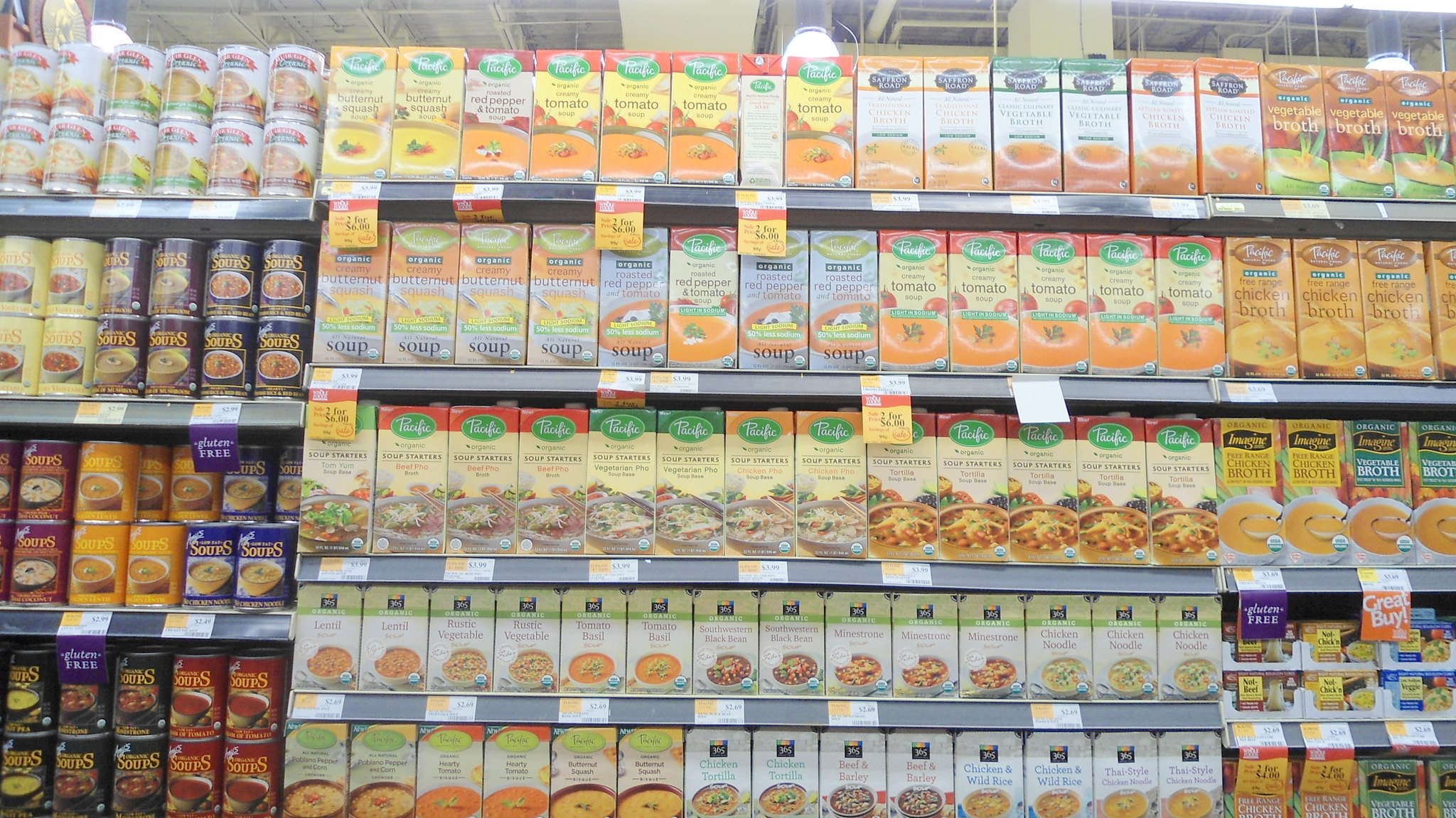The image captures a color photograph of a supermarket aisle dedicated to soups. Dominating the scene are five rows of boxed soups mainly from Pacific Foods, featuring a variety of flavors including butternut squash, tomato, vegetable broth, chicken broth, red pepper, creamy butternut, and other smaller, unreadable flavors. The shelf also holds a selection of boxed soups from the Imagine brand and 365 Organic brand, with flavors like chicken noodle, minestrone, southwestern black bean, tomato basil, rustic vegetable, lentil, chicken tortilla, beef and barley, chicken, and wild rice. Flanking this central display are shelves of canned soups, with labels in various colors—red, brown, blue, yellow, and white—though the specific manufacturer names are unclear. The supermarket setting is accentuated by visible industrial elements, such as roof beams and air conditioning pipes, giving a sense of the typical, functional architecture of a grocery store. Some sale cards are attached to the shelves, highlighting discounts but the exact details are unreadable.